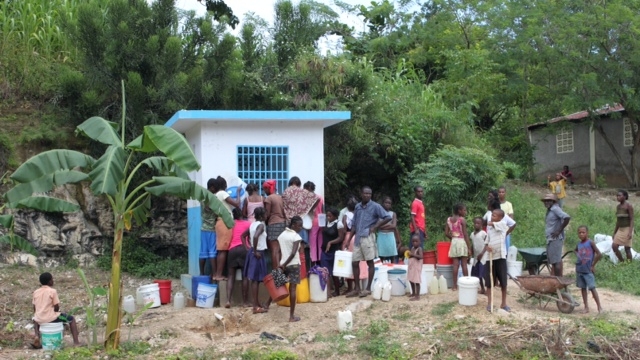In this daytime outdoor photograph, a large group of people, primarily young individuals of African descent, are gathered around a small, white building with a blue slanted roof and a blue grid window. The scene is set against a backdrop of lush, green tropical trees, including a small palm tree near the left. The surrounding area is a mix of green grass, shrubs, and a brown dirt walkway. The people, dressed mostly in shorts and t-shirts, are lined up, many carrying large jugs, buckets, and wheelbarrows, suggesting they are waiting to collect something, likely water. Children and adults alike are mingling around the building, with one child wearing a peach shirt sitting on a labeled white bucket near the palm tree. Off to the right, there appears to be a gray building with rectangular windows, further emphasizing the modest, rural setting.